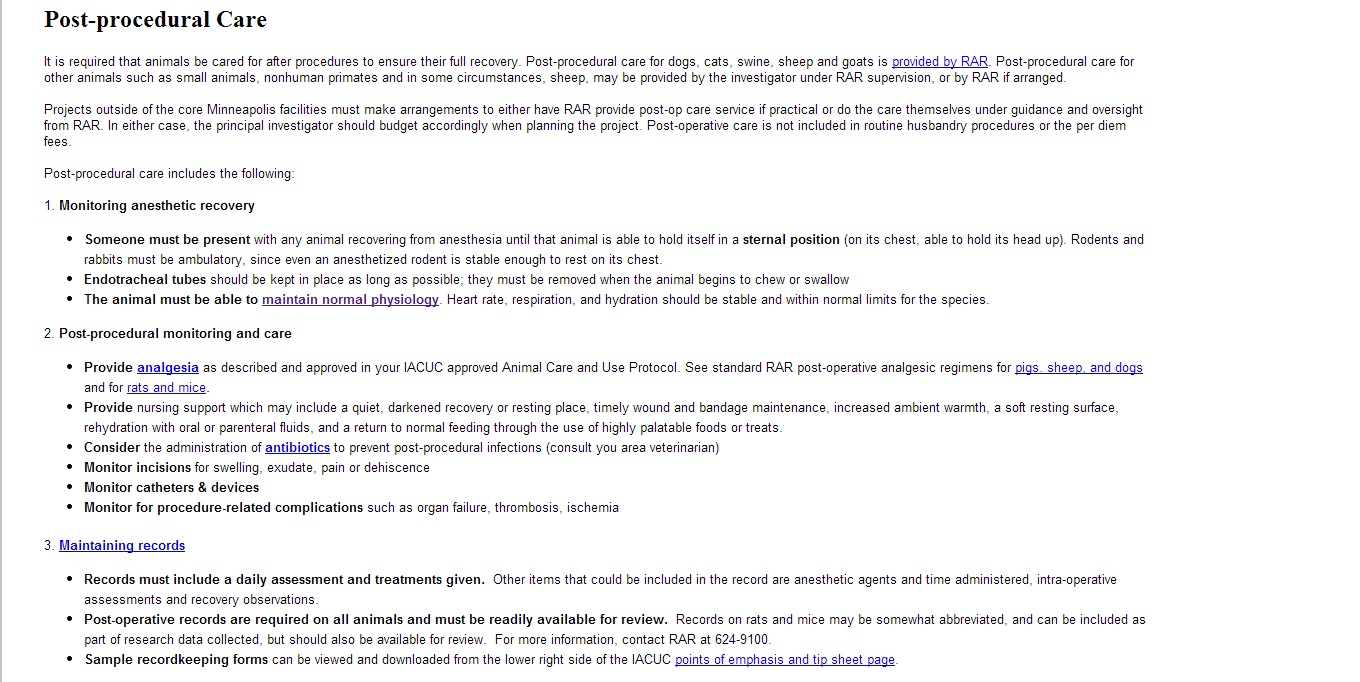**Detailed Caption:**

The image captures a comprehensive list detailing post-procedural care recommendations for various animals. The list emphasizes the importance of ensuring full recovery through meticulous post-procedural care. The text highlights that for dogs, cats, swine, sheep, and goats, post-procedural care is provided by the Research Animal Resources (RAR), with a clickable, underlined link marked in blue for further information.

For other animals, such as small animals, non-human primates, and in some cases, sheep, the care may either be managed by the investigator under RAR's supervision or by RAR itself if prior arrangements are made. Additionally, it mentions that projects conducted outside the Minneapolis facilities need to either arrange for RAR to provide post-operative services where feasible or undertake the care themselves, while adhering to RAR's guidance and oversight.

The document also outlines specific protocols for monitoring anesthetic recovery, listing three bullet points:
1. Presence of a person is required.
2. Endotracheal tubes should be retained as long as possible.
3. The animal must maintain normal physiological functions.

Further down, the document addresses post-procedural monitoring and care with six detailed bullet points, followed by a section on maintaining records, which consists of three bullet points.